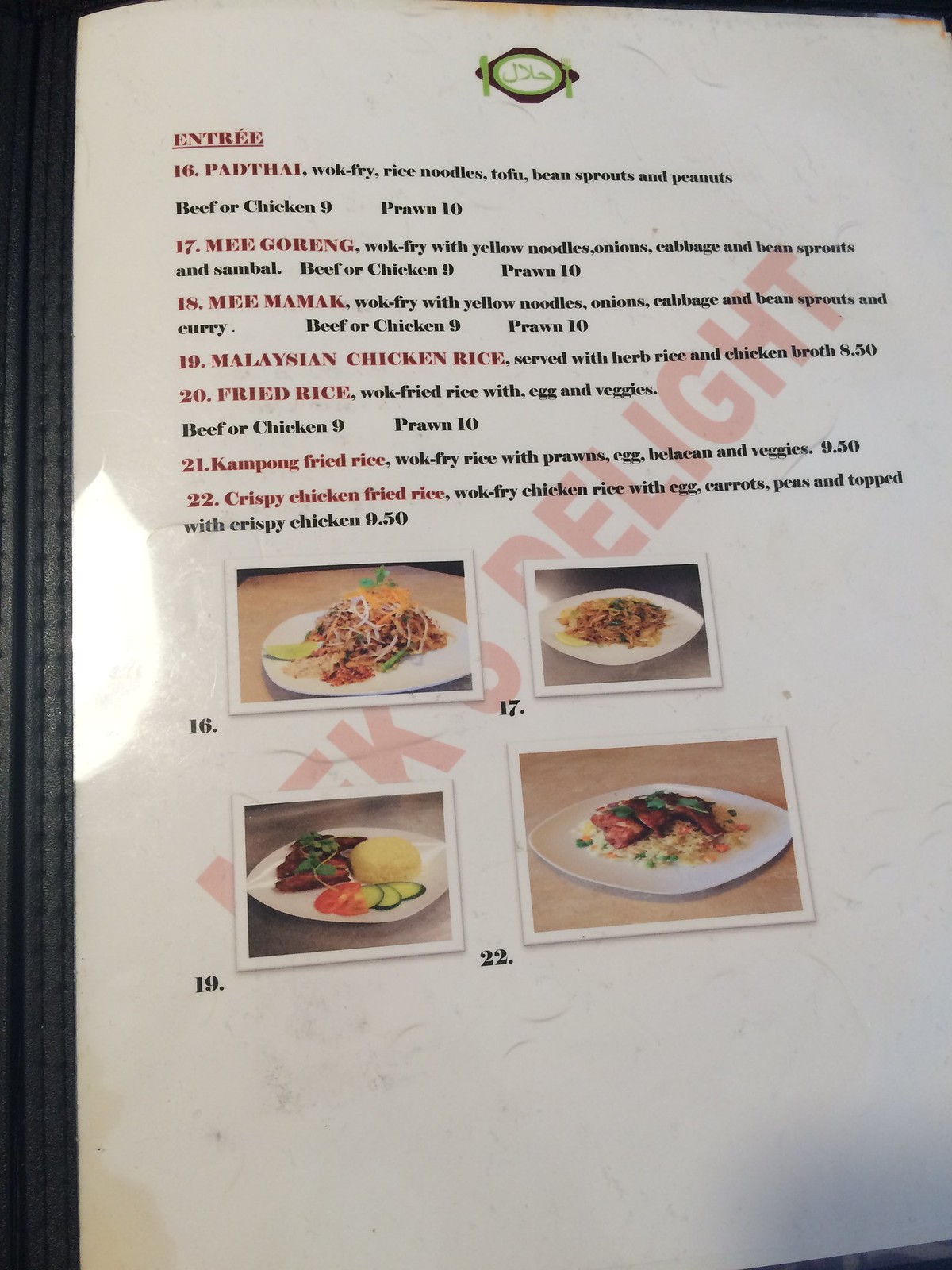Photograph of a menu housed in a protective sleeve, bound on the left side with a sleek black strip that appears to be made of satin or plastic. The laminated menu is reflective, capturing subtle light and shadow on its left side. Despite the protective sleeve, there are visible smudges and marks on the surface, including red or orange specks towards the top. Predominantly white, the menu features a green circular design of a fork, knife, and plate encased within a brown diamond border. At the center, "Delight" is prominently printed across the menu. The lower section displays four images of plated dishes on white plates, highlighting entrees such as Pad Thai with wok-fried rice noodles, tofu, bean sprouts, and peanuts, as well as Mee Goreng with wok-fried yellow noodles, onions, cabbage, and bean sprouts, indicating an Asian culinary theme.